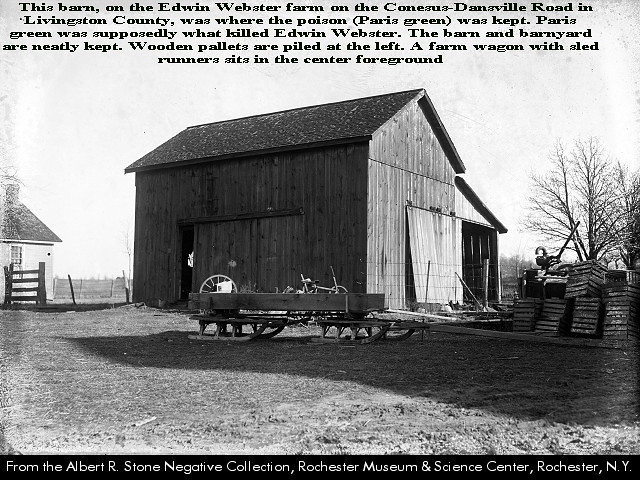This black and white photograph, from the Albert R. Stone Negative Collection at the Rochester Museum and Science Center, Rochester, New York, depicts the barn on the Edwin Webster farm located on the Kinesis-Dansville Road in Livingston County. The barn, where the poison Paris Green—believed to have killed Edwin Webster—was kept, showcases a neatly kept barnyard. The sliding door of the barn is slightly ajar, revealing a glimpse inside. Wooden pallets are piled up on the left side of the barn, while a farm wagon with sled runners is prominently positioned in the center foreground. To the right, part of a house or possibly a chicken coop is visible, enhancing the rustic, historical setting.